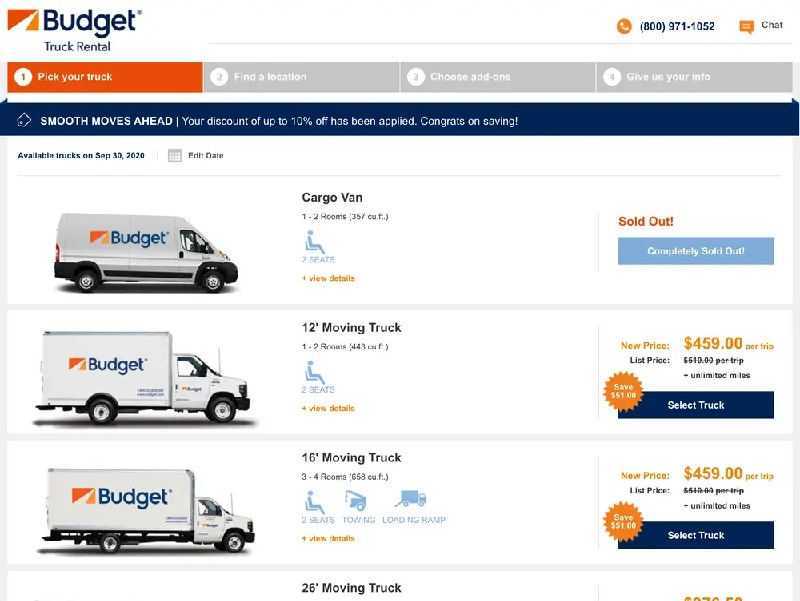On the Budget Truck Rental website, the top banner prominently displays the company name "Budget Truck Rental" in blue text, accompanied by the Budget Truck Rental logo. The logo is a distinctive design featuring an orange square with two orange sides and a white bottom. To the right of this header, the website provides the company's phone number and a chat option for customer support. 

Below the header, there is a navigation bar with the steps: "Pick Your Truck," "Find a Location," "Choose Add-Ons," and "Give Us Your Info." Farther down, a highlighted message reads, "Smooth moves ahead. Your discount of up to 10% off has been applied. Congrats on saving." This message signifies a promotional discount.

The webpage then lists the available truck rentals for September 30th, 2020:

1. **Cargo Van**: Suitable for moving 1 to 2 rooms, this option is currently sold out.
2. **12-Foot Moving Truck**: Capable of accommodating 1 to 2 rooms and equipped with two seats. Priced at $459 per trip with unlimited mileage. Users can select this truck for their move.
3. **16-Foot Moving Truck**: Designed for moving 3 to 4 rooms and also has two seats. It is available for $459 per trip and offers unlimited mileage.
4. **26-Foot Moving Truck**: This option is listed without detailed information such as size, price, or additional features, other than noting its availability.

Images accompany each truck option, except for the 26-foot moving truck, which lacks a visual representation and detailed description.